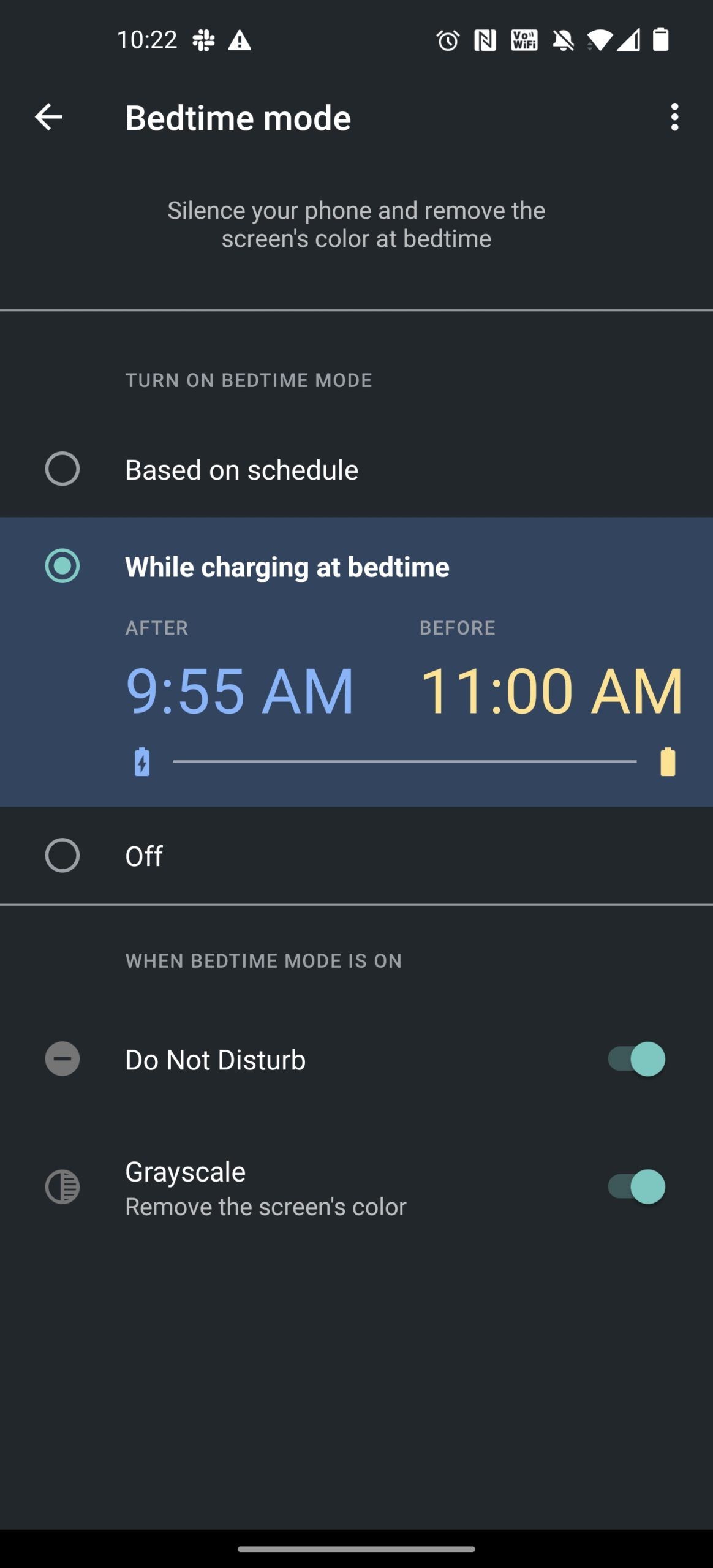This is a detailed screenshot from a smartphone displaying the "Bedtime Mode" settings interface. At the very top of the screen, the time is indicated as 10:22. To the right of the time, there is an alert symbol followed by a triangle icon, with additional options visible beyond these indicators. The signal strength is nearly full, and the battery is almost fully charged.

Immediately below this top bar, there is a back arrow on the left and the text "Bedtime Mode" in white on a black background. To the right of the text are three vertical dots, indicating more options.

The main section of the screenshot begins with the instruction: "Silence your phone and remove the screen's color at bedtime." Below this, there is an option to turn on Bedtime Mode, displayed with a circle that is unselected, next to the text "Based on schedule."

The next setting option is highlighted in a blue box with a marked circle, indicating it is selected. The bold text reads: "While charging at bedtime."

Following this, the interface details a schedule: "After 9:55 AM" displayed in blue, and "Before 11 AM" displayed in orange.

Further down, there is an option labeled "Off," which is unselected.

When Bedtime Mode is active, two options are shown, both of which are selected. The first option, "Do not disturb," features a symbol of a circle with a minus sign. The second option, "Grayscale," includes a half-filled circle icon and the description "Remove the screen's colors."